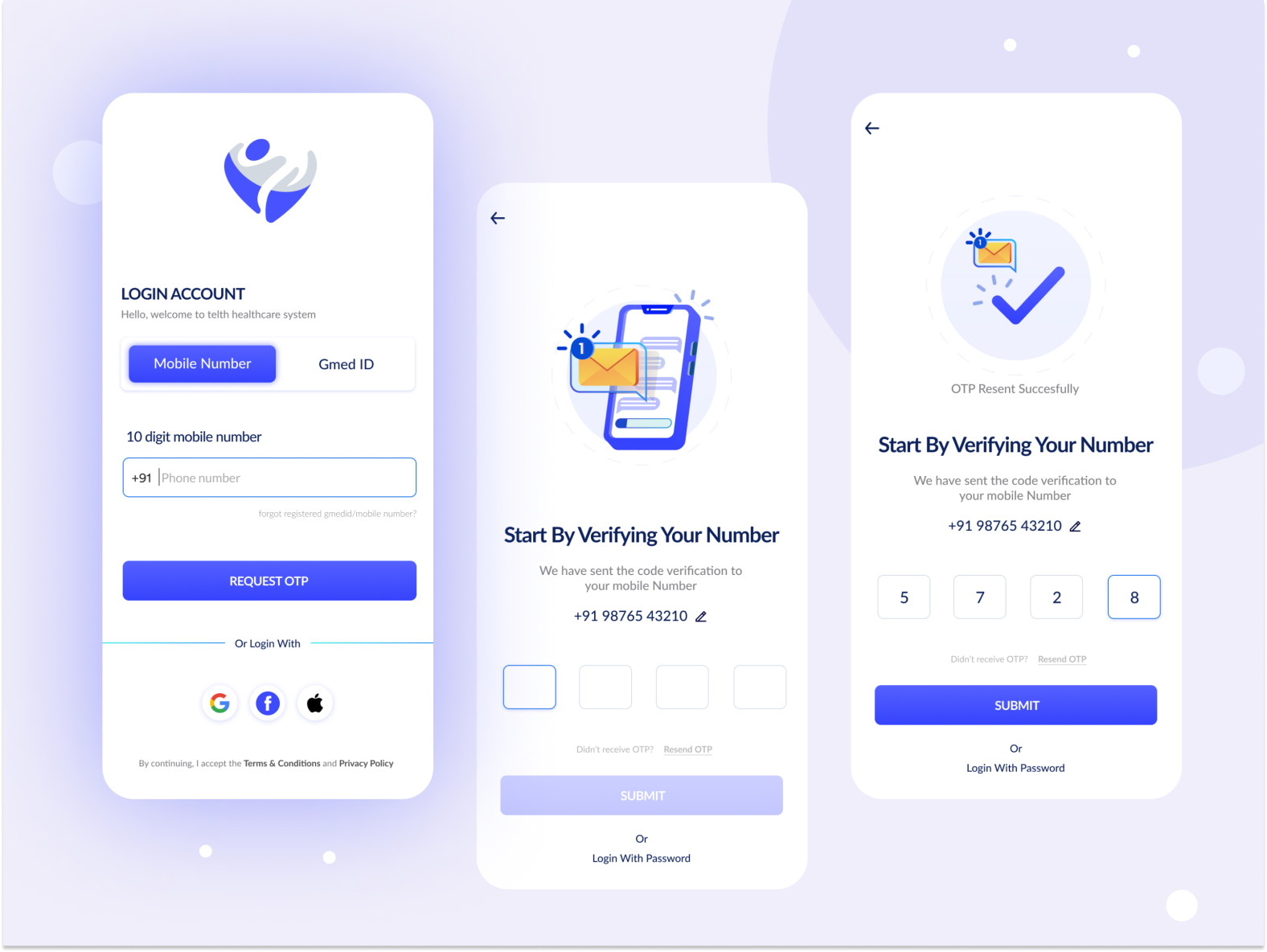In this image, a web page displays a streamlined, three-step process for user authentication. The first screen prompts users to either log in or create an account using a 10-digit mobile number, with an additional option to request a one-time password (OTP) for enhanced security. The second screen guides users through the verification of their mobile number, necessitating the entry of the received OTP. The third and final screen requires the user to input the OTP to complete the authentication process, thereby ensuring a secure and verified login experience.